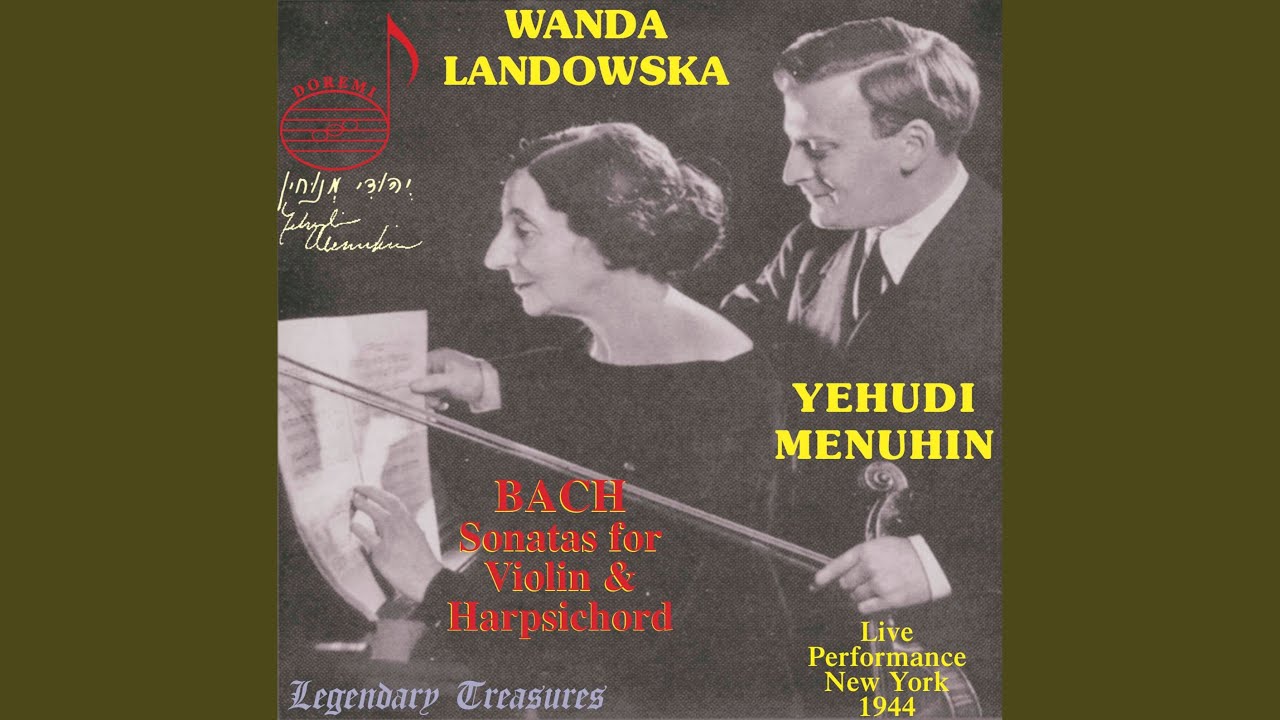The image showcases a vintage black and white poster of a live musical performance by Yehudi Menuhin and Wanda Landowski, titled "Legendary Treasures." The poster prominently displays the words "Bach Sonatas for Violin and Harpsichord" at the bottom left. Yehudi Menuhin, identified by his name across his midsection, is dressed in a suit with a white shirt and black tie while holding a partially obstructed violin, his focus on a sheet of music. On the right, Wanda Landowski, with short curly hair and a distinct profile featuring a long nose, is also engrossed in the sheet music. Her name is positioned above her in yellow. The bottom right of the poster states, "Live Performance, New York, 1944," indicating the historical context. The arrangement of musical elements and the stylized title in cursive likely suggest this is a cover for a CD or record capturing this iconic performance.